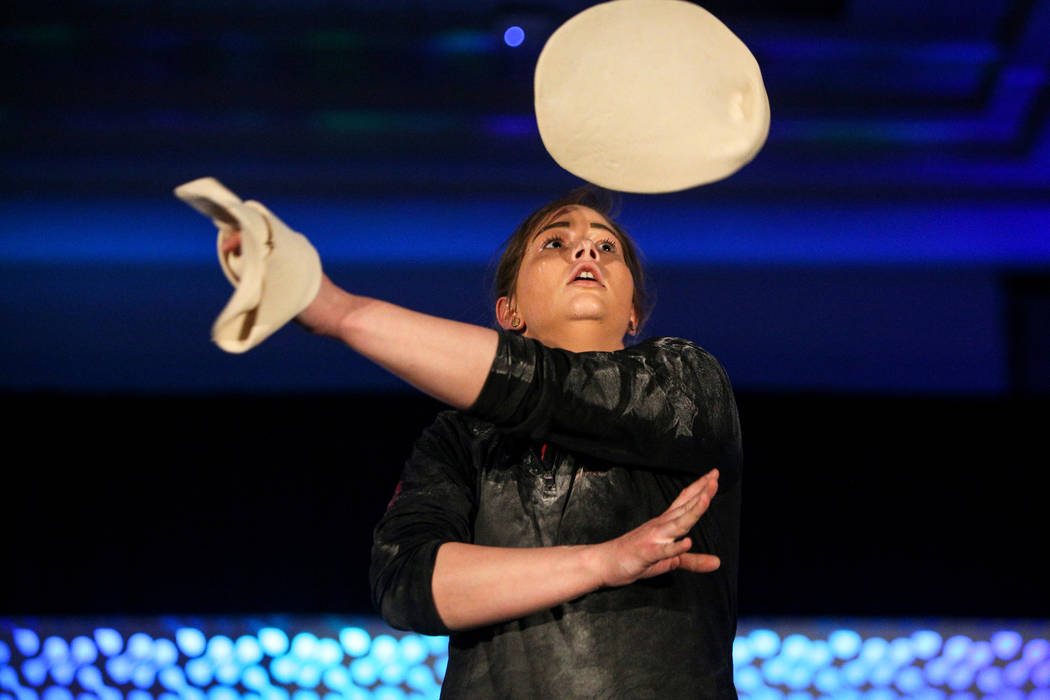In the image, a woman with brown hair, wearing a black flour-dusted shirt and earrings in each ear, is caught in the midst of a dynamic motion that suggests dancing or performing. She is the focal point, positioned centrally with her head slightly tilted upwards, revealing her nostrils. Her left arm is extended towards the left side of the image, holding a white or cream-colored object, possibly an ankle brace or dough. Her right arm crosses her chest, angled towards the left. Above her head floats a circular, light brown or cream-colored object resembling a pizza crust or dough ball. The backdrop is dark, accented by blurred blue and light blue dots near the bottom, giving an impression of clustered lights, possibly indicating a concert or performance setting.